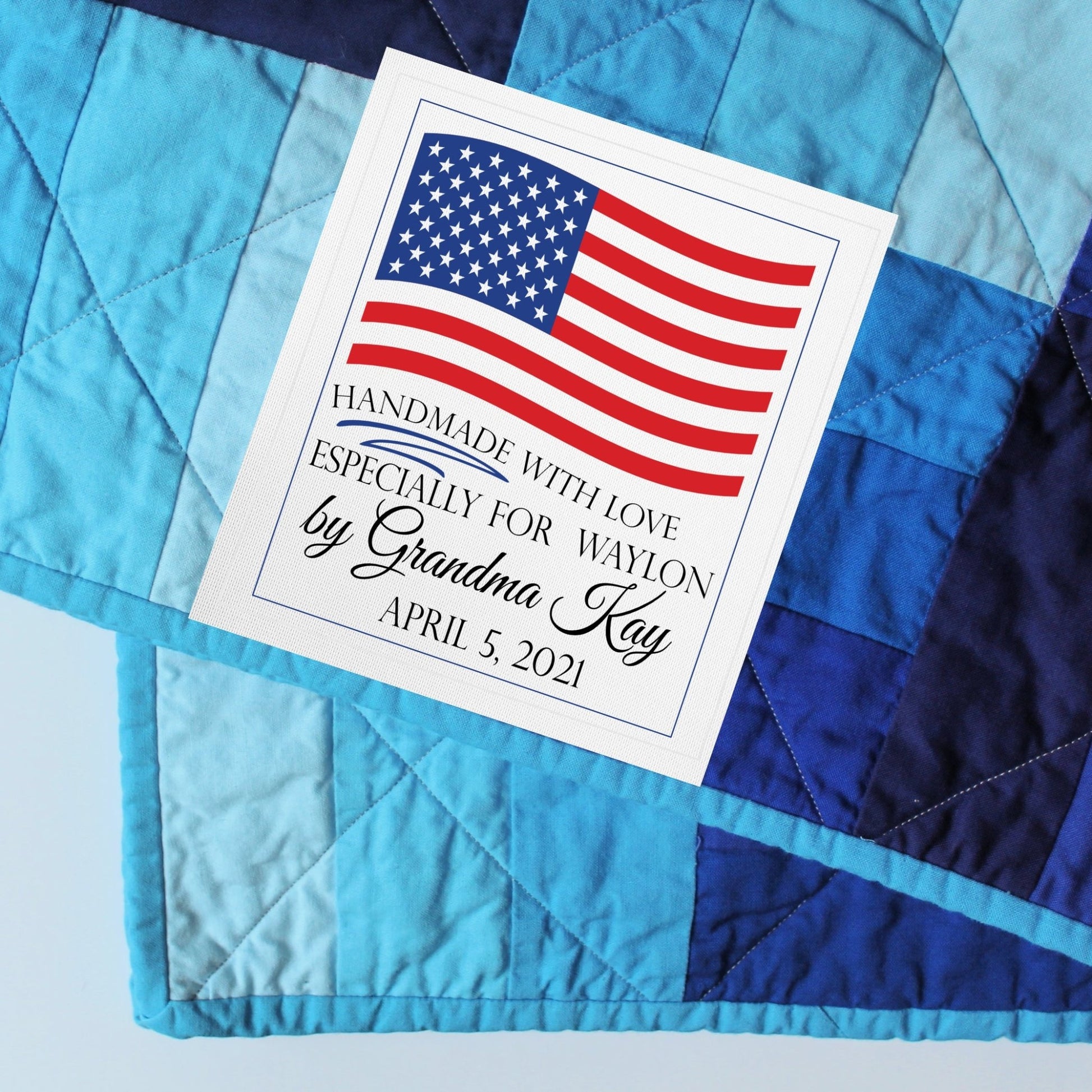This detailed image captures the bottom portion of a vibrant quilt made up of an assortment of blue patches, displaying hues from turquoise and light blue to royal blue, navy, and electric blue. The quilt's texture reveals meticulous stitching between these colorful sections, characteristic of a patchwork design. A prominent, square-shaped white label is affixed to the quilt, centrally positioned in the photograph. The label, bordered in blue, features a red, white, and blue American flag at the top. Beneath the flag, in black cursive and regular font, the text reads, "Handmade with love especially for Waylon by Grandma Kay, April 5th, 2021." The quilt’s edge shows a light blue, almost turquoise border, adding to its intricate detailing and craftsmanship. The overall presentation exudes warmth and personalized care, indicative of a treasured handmade creation.